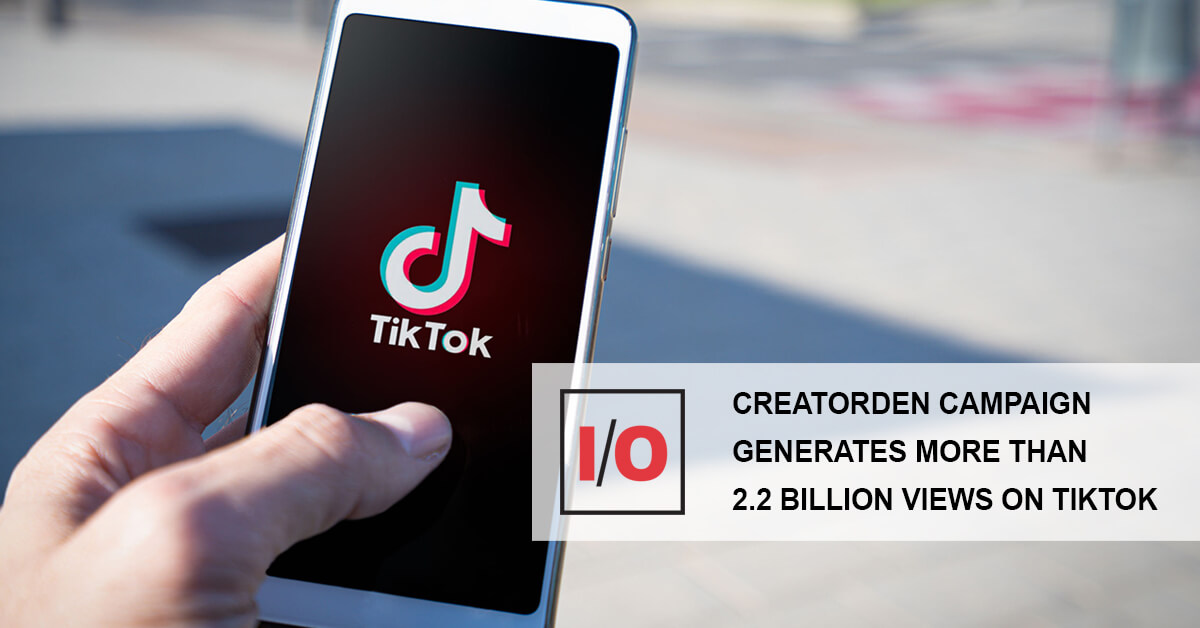In this image, a person is holding a smartphone in their left hand, displaying the TikTok app on the screen. The fingers are positioned behind the phone, with the thumb on the front, securing the device. The TikTok icon is prominently visible against the recognizable black background of the app. Beside the icon, a notification reads "1/0," both numbers highlighted in red and enclosed within a black-outlined box.

Additionally, there's a notable rectangular banner on the screen announcing a significant milestone: "Creator Den campaign generates more than 2.2 billion views on TikTok." Behind the phone, the background is blurred, but it appears to depict a playground-like area with a white floor and vibrant pink, yellow, and blue colors scattered on the ground. The phone casts a distinct blue shadow underneath it. Two vertical poles can be seen near the pink area, and a small black dot is noticeable in the upper left-hand corner of the image.